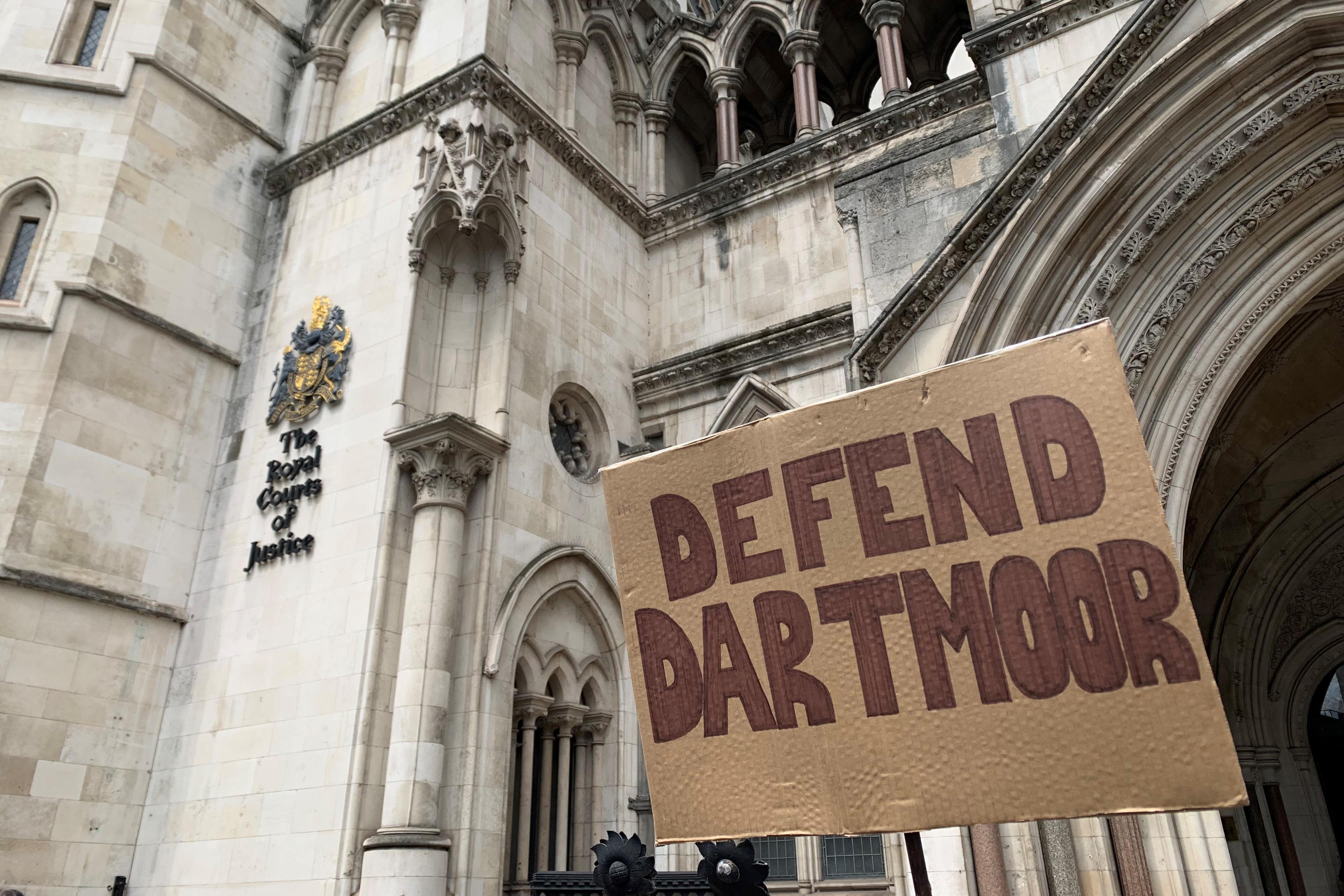The image captures the impressive facade of the Royal Courts of Justice, a large and elaborate Gothic-style building constructed from bricks in various shades of tan, light yellow, and white. The left side of the building features a prominent crest, beneath which the black letters spell 'The Royal Courts of Justice.' The architecture showcases intricate details, with large arches and columns adding to its grandeur, resembling the ornate style of a cathedral. On the right side of the frame, a segment of an elaborate archway is visible, partially cut off. Directly in front of this archway stands a handmade cardboard sign with red, fully filled-in bubble letters that read "DEFEND DARTMOOR." The photograph, taken during the daytime, highlights the juxtaposition of the formal, historic building with the informal protest sign.